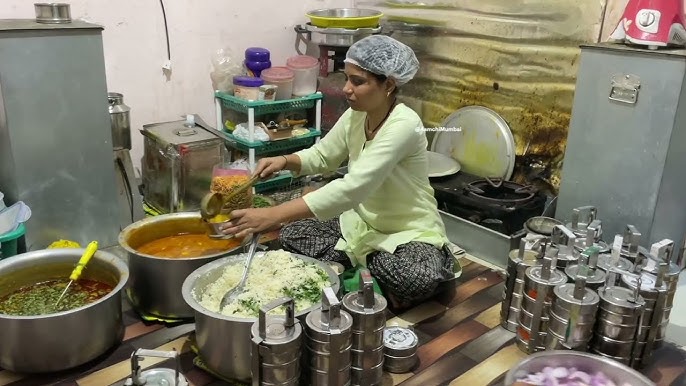In an industrial kitchen, a woman is seated cross-legged, preparing food. She is wearing a mint green shirt, a white hairnet, and black pants with white speckles. With a large spoon, she ladles reddish stew into a small cup over a large pot. Surrounding her are three large pots: one with white rice mixed with greens, another with a reddish soup topped with green vegetables, and a third with a brownish soup. The image also shows a silver bowl filled with sliced purple onions. The kitchen is cluttered with numerous metal canisters and bowls and appears unclean, with walls stained brown and yellow from extensive cooking. A silver storage unit with a red item on top is also visible in the background.